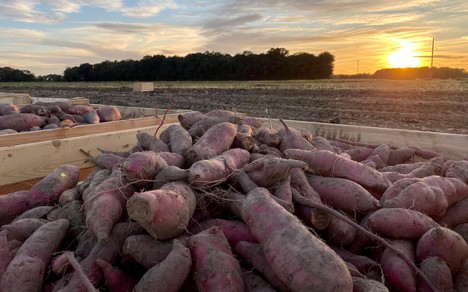The photograph captures a recently harvested farm field with distinct brown ruts running from the top left corner to the mid-right side, indicating the passage of machinery. In the foreground, two large wooden crates, crafted from boards, are brimming with reddish-brown, oblong root vegetables, presumably sweet potatoes given their color and shape. Another similarly filled crate is visible further into the field. The harvested field appears barren, with a neighboring field that seems to have been mowed visible in the midground. Beyond the fields lie several clusters of dark green trees, their leaves darkened by fading sunlight. Metal electric poles stand in the distance, lining what appears to be a roadway. The scene is set against a backdrop of a dusky sky, where the setting sun in the top right corner casts a yellow glow, creating light gray and blue hues among the clouds.